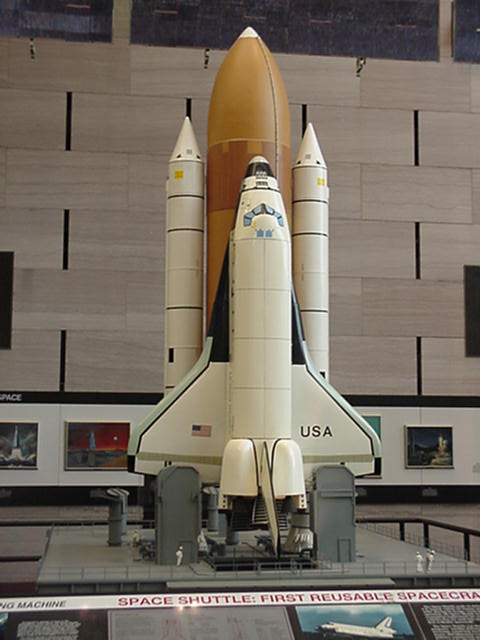The image shows a detailed scale model replica of the United States Space Shuttle, prominently displayed in what appears to be a museum setting, likely an air or space museum. The space shuttle model, complete with its attached launch rockets, stands upright on what resembles a launch pad platform. Its large brown main tank and white rocket boosters with black stripes are accurately depicted, as is the space shuttle itself, which is white with black areas.

In front of the platform is a display stand labeled "Space Shuttle First Reusable Spacecraft," accompanied by photographic and text placards that offer detailed information about the shuttle. Although the text on the placards is too small to read clearly, they contain descriptions and historical data about the spacecraft. Miniature scale models of people positioned around the base of the shuttle provide a sense of scale, emphasizing the enormity of the spacecraft.

The backdrop of the exhibit comprises a wall designed with a stone-like pattern, adorned with various photographs of space shuttle launches, adding contextual depth to the display. The meticulous details of both the model and its informative surroundings create an immersive and educational visual experience.